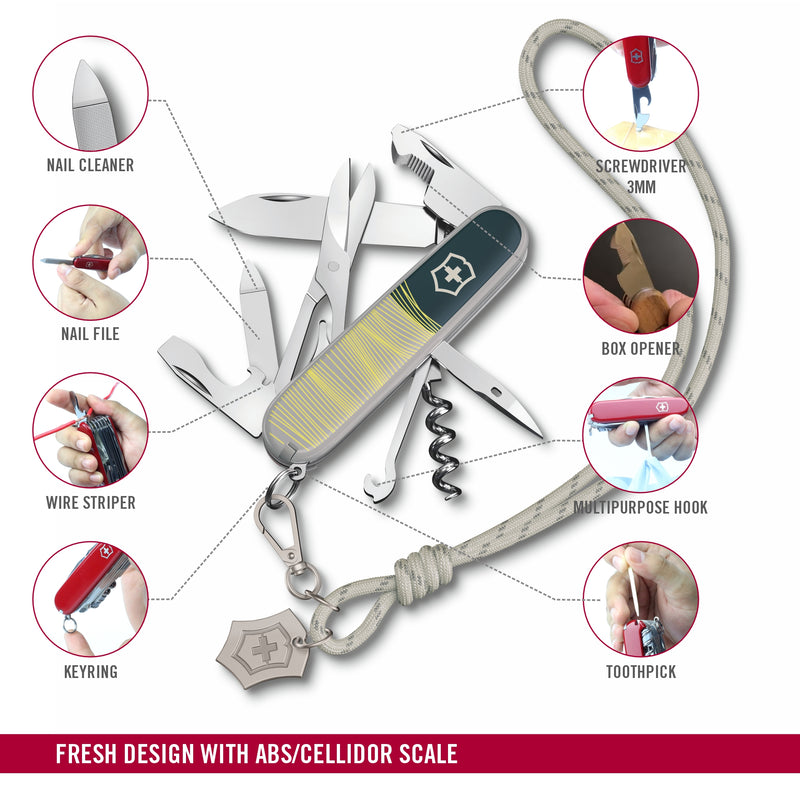The image is an advertisement or infographic showcasing a Swiss Army knife with a fresh design and ABS Cellidor scale. The background is a clean white, overlaid with a detailed layout of the multi-tool knife, featuring a mix of black, tan, white, and silver colors. This long, elongated oval pocket knife prominently displays the iconic Swiss Army insignia—a cross on a shield. Attached to the knife is a sturdy rope lanyard, a mix of gray and white wool, extending to the upper right-hand corner and functioning as a keychain. 

The knife itself is sectioned into various tools, each highlighted with descriptive circles and labeled: Nail Cleaner, Nail File, Wire Stripper, Key Ring, Screwdriver 3mm, Box Opener, Multi-Purpose Hook, and Toothpick. The top part of the knife, in the upper right-hand corner, includes a saw blade tool specifically identified as the Box Opener, also serving as a Screwdriver 3mm at its tip. Other notable tools include a short knife, a hook labeled as Multi-Purpose Hook, and a cutout base labeled as Wire Stripper. The bottom left hosts a ring named the Key Ring, important for its multifunctionality. These tools reflect a tight integration of utility in a compact design. 

The advertisement text emphasizes "Fresh Design with ABS Celador Scale," positioned at the bottom within a red stripe with white fonts. This central visual display aims to highlight each functional component, allowing for easy identification and appreciation of the Swiss Army knife's versatility and modern design elements.